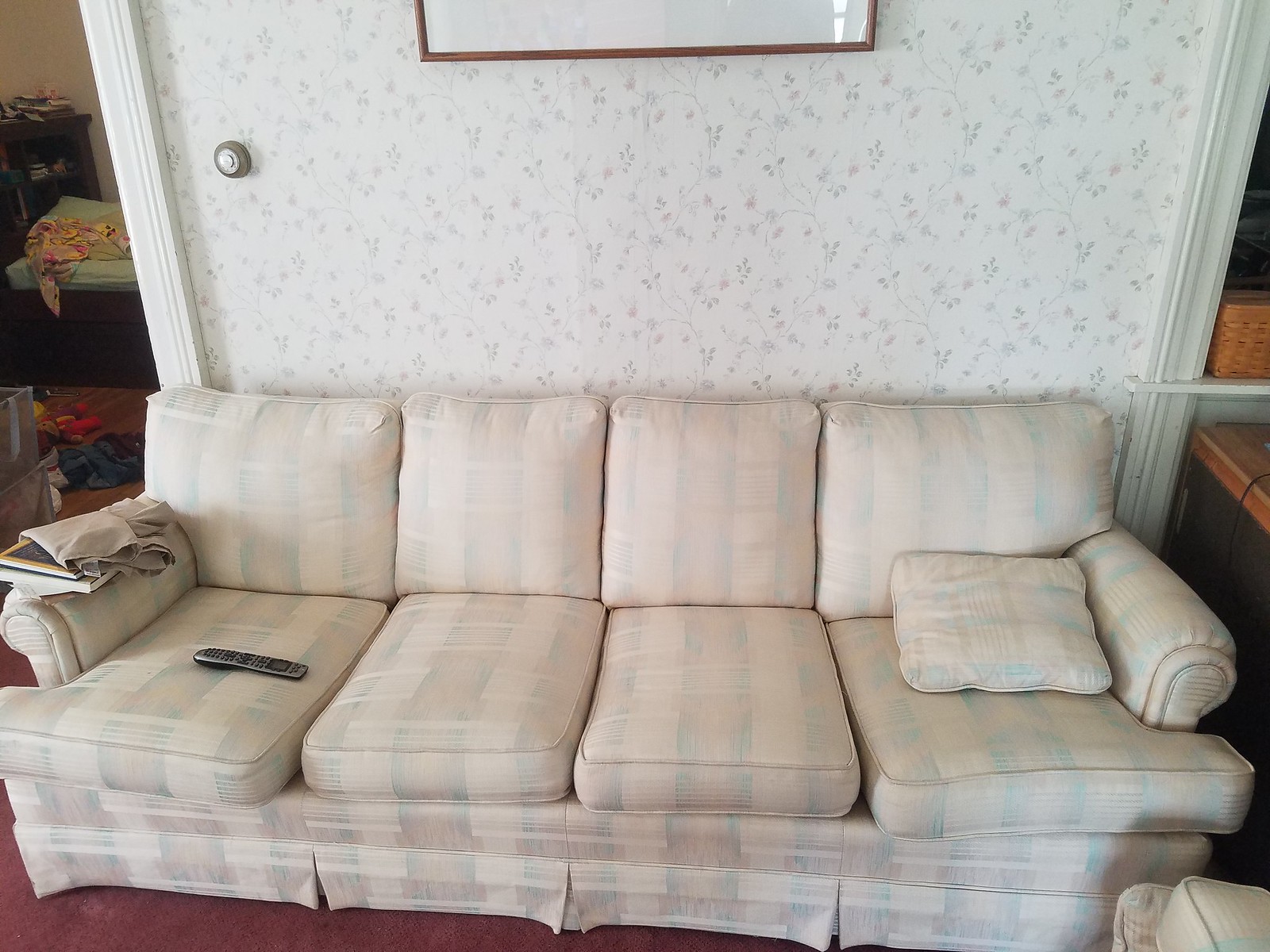This photograph captures a light off-white couch with a subtle, faded plaid pattern of blue and pink stripes, set against a backdrop of a floral wallpapered wall. The couch, featuring four seat and back cushions, occupies a space in front of a maroon carpet. A single throw pillow, matching the couch’s pale color scheme, rests on the right side. Adding to the scene's everyday realism, a black remote control sits on the far left cushion, and a couple of books and a folded piece of laundry lie on the left armrest. The background reveals a doorway on the left, opening into a messy bedroom with clothes scattered on the bed. A second doorway is visible on the right. The wall above the couch is adorned with a circular thermostat on the left side, and the bottom edge of a wooden-framed white painting is visible at the top of the photo.